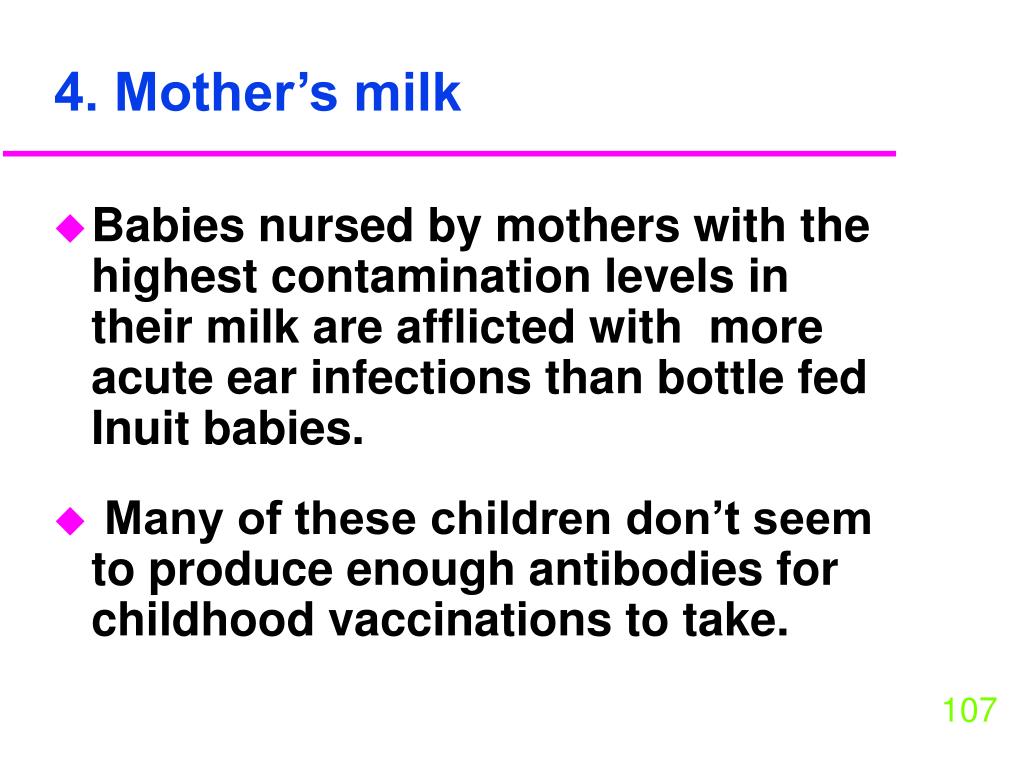The image depicts a simple, text-based informational slide, likely the fourth in a PowerPoint presentation. The slide features a title at the top, "Mother's Milk," written in blue text with the number 4 prefacing it. Directly beneath the title runs a bright magenta (or purple) horizontal line. Below the line, there are two bullet points, each marked by a magenta diamond shape. The text of the bullet points is in black Arial font and reads:
1. "Babies nursed by mothers with the highest contamination levels in their milk are afflicted with more acute ear infections than bottle-fed Inuit babies."
2. "Many of these children don't seem to produce enough antibodies for childhood vaccinations to take."

The background of the slide is plain white, and at the bottom right corner, the number 107 is displayed in small lime green text. This minimalistic slide contains no graphic images or additional design elements.